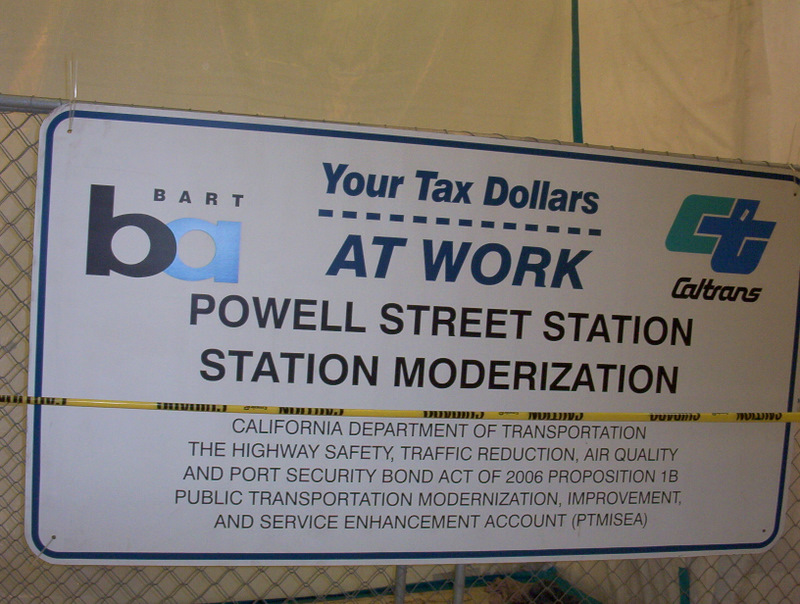In this photograph, a chain-link fence holds a large, rectangular metal sign attached with metal clips. The sign features a white background and a thin blue border, with text in both blue and black. At the top middle, in blue text, it reads "Your Tax Dollars," followed by a dotted line, and then below in larger blue letters, "At Work." Below this, in black text, is "Powell Street Station" and "Station Modernization." The upper right corner of the sign displays the interconnected green and blue logo of Caltrans, with "Caltrans" written beside it. On the upper left corner, there is a BART logo, with "BART" in black and a smaller "b" in black and "a" in metallic blue next to it. Further text at the bottom center reads: "California Department of Transportation," followed by "The Highway Safety, Traffic Reduction, Air Quality, and Port Security Bond Act of 2006," and lists "Proposition 1B," "Public Transportation Modernization, Improvement, and Service Enhancement Account (PTMISEA)." The background of the scene is filled with a cream-colored cloth, visible through the metallic fence.